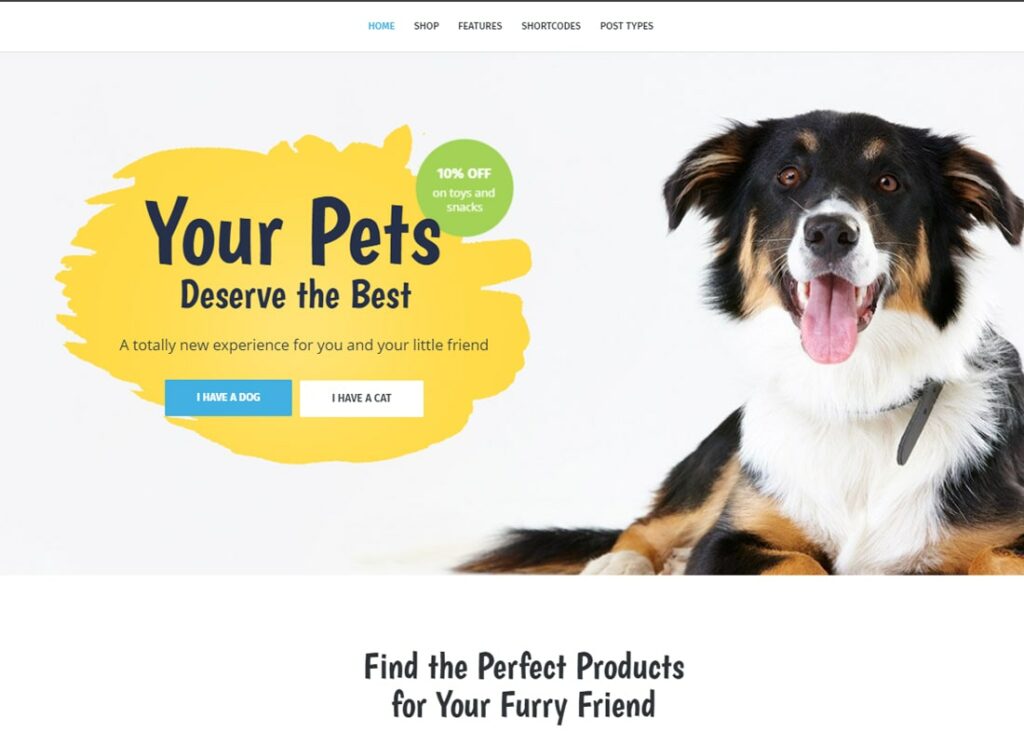The screenshot captures the homepage of a pet-centric website designed for pet owners to shop for their furry friends. At the top of the page, there is a navigation bar with tabs labeled "Home," "Shop," "Features," "Shortcodes," and "Post Types." Below the navigation bar, the main section of the page features a vibrant image of a Collie in black, orange, and white colors, sitting on the floor. The Collie wears a collar and looks eagerly at the camera, exuding a lively and friendly demeanor.

To the left of the Collie's image, there is a promotional banner that reads, "Your pets deserve the best – Enjoy 10% off on toys and snacks." This section emphasizes a new experience for pet owners and their pets. Below the promotional message, there are two clickable buttons labeled "I have a dog" and "I have a cat," each accompanied by a yellow paw print icon.

Additionally, a highlighted call-to-action at the bottom of the screenshot encourages users to "Find the perfect products for your furry friend." This further suggests the website is dedicated to providing a variety of treats, food, and other products for both dogs and cats, and possibly other types of pets. Overall, the website appears to be a go-to destination for pet owners looking to spoil their pets with high-quality items.